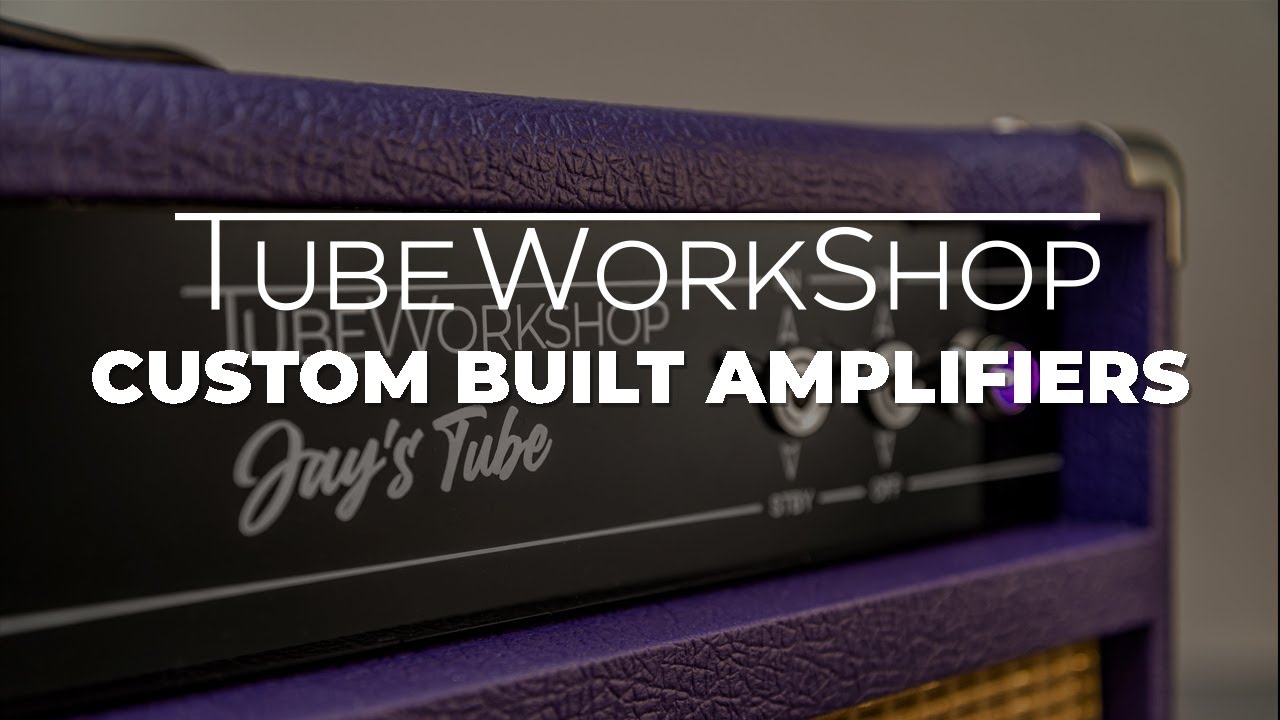This horizontally oriented photograph showcases a close-up of a custom-built amplifier from Tube Workshop. Dominating the foreground, bold white text proclaims "Tube Workshop Custom Built Amplifiers" in large, thin letters, while smaller, fatter letters state "Jay's Tube." The amplifier itself is encased in either indigo or navy blue leather with metal corners and a tan-colored screen portion emerging at the bottom. The amplifier features silver metal knobs and switches. The background is a plain, dark gray wall, which draws attention to the detailed craftsmanship and branding of the amplifier.